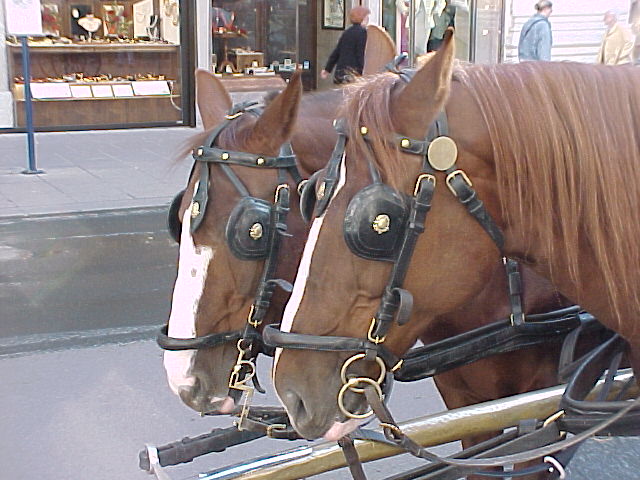This color photograph, taken outdoors, captures a detailed view of two brown horses with white stripes down the fronts of their faces, likely harnessed to pull a carriage. The image, oriented horizontally, shows the horses from the front and side, highlighting their black leather harnesses, complete with gold buckles and detailed eye blinders, which allow them to see only straight ahead. The two horses, with brown manes, are positioned in front of a city street lined with stores and shops, including what appears to be a jewelry store, given the mannequins and boxes displayed in the window. In the background, three pedestrians can be seen: a man in a light blue hoodie, another in a light yellow jacket, and a woman in black. A blue street sign can be spotted at the top left corner, adding to the urban setting as the horses stand on the concrete street.